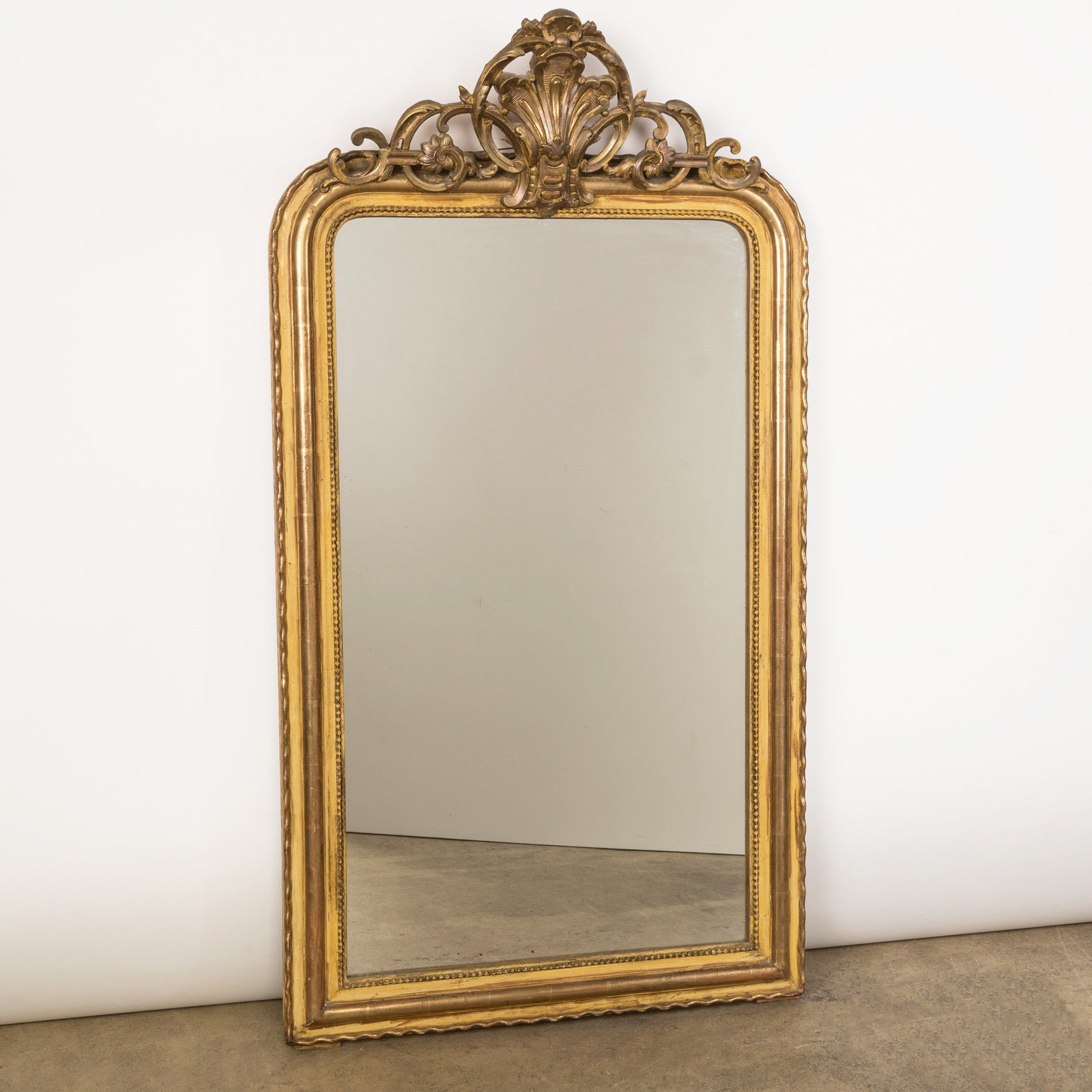The image displays a striking antique-style, full-length rectangular mirror leaning against a plain white wall, set on a brown floor. The mirror's frame is a rich gold color, adorned with intricate detailing and decorative motifs. Particularly standout is the top of the frame, which features an elaborate symmetrical crest incorporating a shell-like design, flanked by swirling leaves and other stylized foliage. The craftsmanship suggests a gilded finish, with inner and outer beaded edges adding texture and depth to the sophisticated border. The rounded top corners blend into the opulent framework, which includes loops, hoops, and knot-like patterns enhancing the visual richness. The mirror's glass is clear and reflects another white wall and brown floor, while the frame’s slightly aged appearance adds to its vintage charm, evocative of the lavish design sensibilities of the 18th or 19th century.